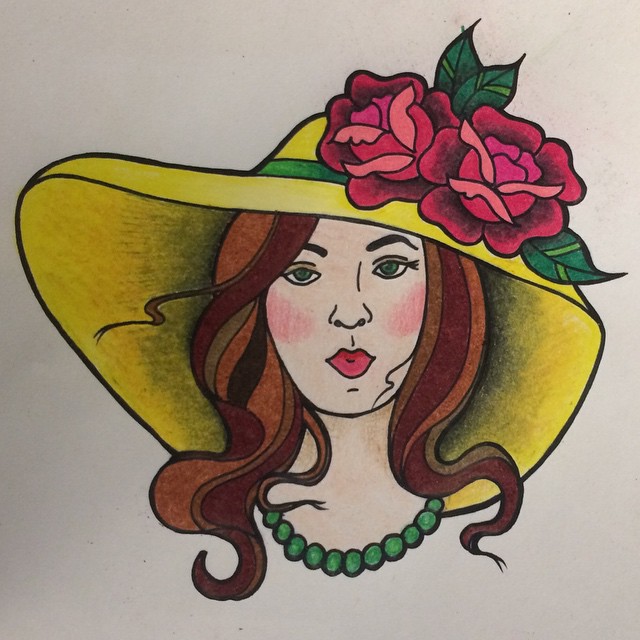This detailed, color illustration on white paper portrays a young woman gazing directly at the viewer. She has long, flowing auburn hair, striking blue eyes, and features enhanced with rosy cheeks and full red lips. Adorning her head is a wide-brimmed, floppy yellow hat, accented with a green hatband. Adding a touch of vivid elegance, two fully-bloomed bright red roses decorate the right side of the hat, accompanied by sprigs of green leaves that extend above and to the bottom right of the roses. Completing her ensemble, the woman wears a green, beaded necklace. The image is devoid of any text, animals, buildings, signs, or motorized vehicles, focusing the viewer's attention solely on the detailed portrait of the woman.